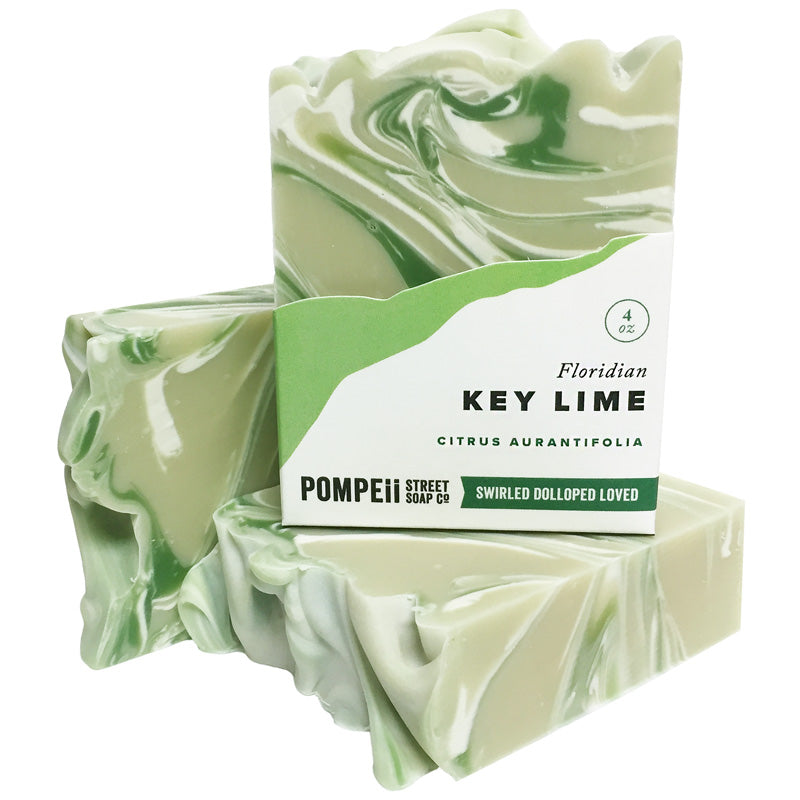This image features an artful arrangement of three bars of handmade soap against a white backdrop. The soap bars have a distinct look with textured swirls in shades of green and white mixed within a beige base. The bar in the foreground is wrapped in a label that reads "Floridian Key Lime, 4 ounces, Citrus Arantifolia." The packaging is white with a green and white rendering of the soap, and the brand name "Pompeii Street Soap Company" is prominently displayed. The packaging also includes a green ribbon design that says "Swirled, Dolloped, Loved." The labeled bar is standing vertically atop another bar lying flat, and a third bar is positioned behind, partially obscured by the front two. The top of the bars is jagged as if broken, adding to the handmade aesthetic.